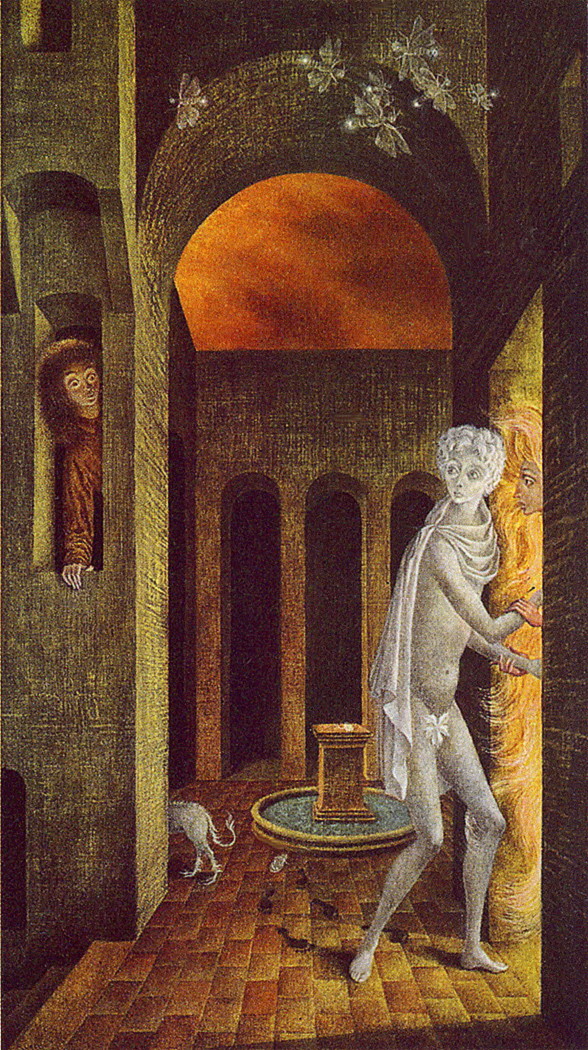This image presents a medieval-style, two-dimensional painting in earthy tones of gold, orange, brown, and yellow. At the center of the composition, a ghostly white figure stands prominently, resembling a human statue with dark eyes, short curly hair, and a fig leaf covering. The figure is naked except for a cape or shawl draped around its neck. It stands in front of one of three doorways with arched tops, which appears to be emitting flames.

The setting appears to be an indoor chapel or hall with a brick floor, a table fountain in the background, and clean structural lines. On the left edge, a figure with long brown hair is seen peeping through a small arched window, hand extended as if reaching out or observing the scene. This character seems to be watching the white figure.

In the right foreground, another person, discernible from their colored face, appears to be dragging or pulling the white figure through the luminous doorway. An additional creature, possibly a cat or dog with two legs and a long tail, peeks around a corner at the bottom of the image, adding to the medieval ambiance of the painting.